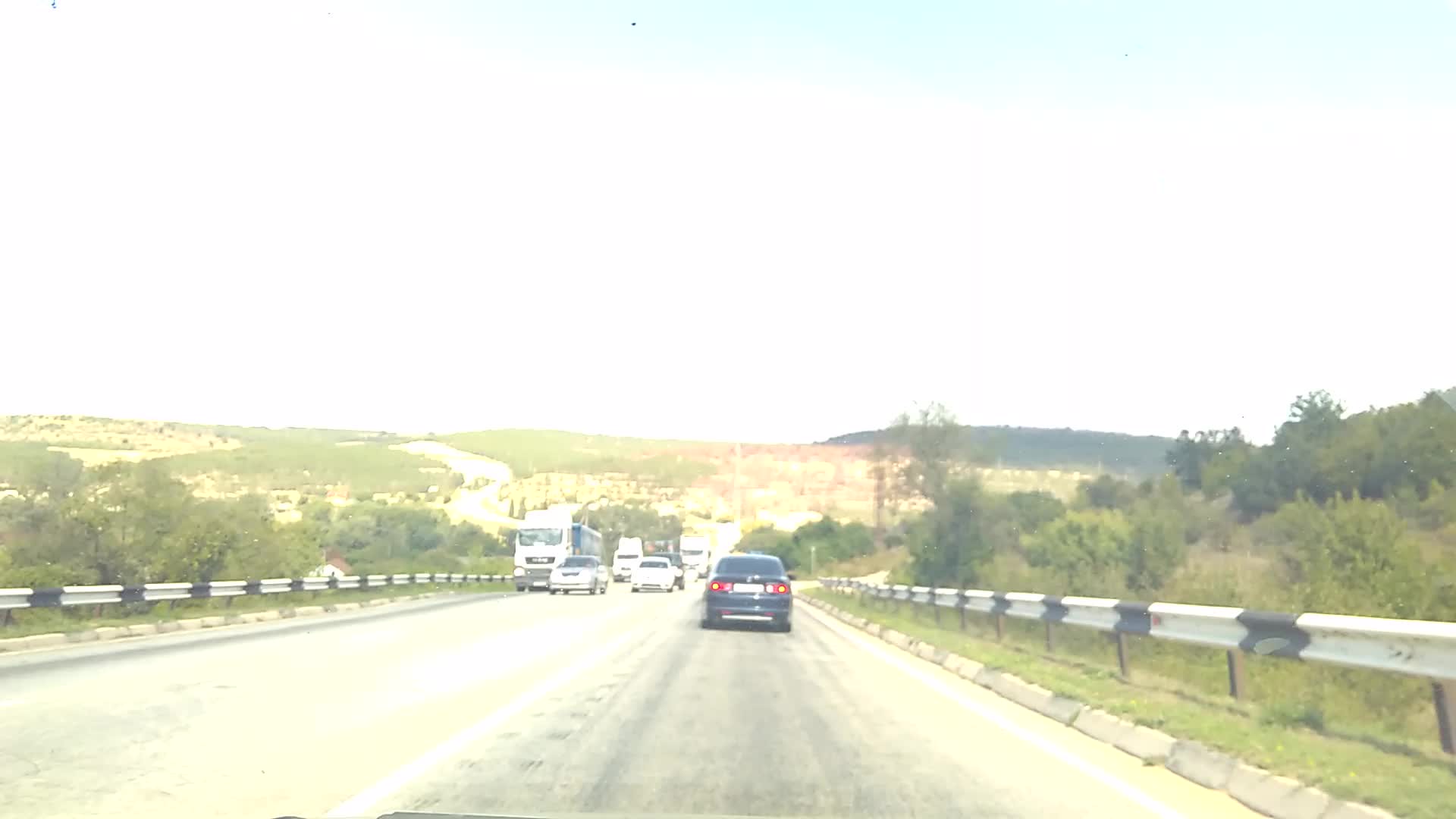This low-resolution, overexposed photograph captures a bustling highway scene. In the right lane moving away from the camera, a dark single-passenger vehicle is prominently visible. Heading toward the camera in opposing lanes are various vehicles, including highway trucks and a bus, contributing to the moderate traffic. The background reveals a gently sloping small hill, sporadically dotted with trees and bushes, providing a hint of natural landscape. The sides of the highway are lined with scrubby bushes, indicating a well-traveled and somewhat weathered road. Overhead, the sky appears gray with patches of blue peeking through, adding to the overall muted tone of the image.